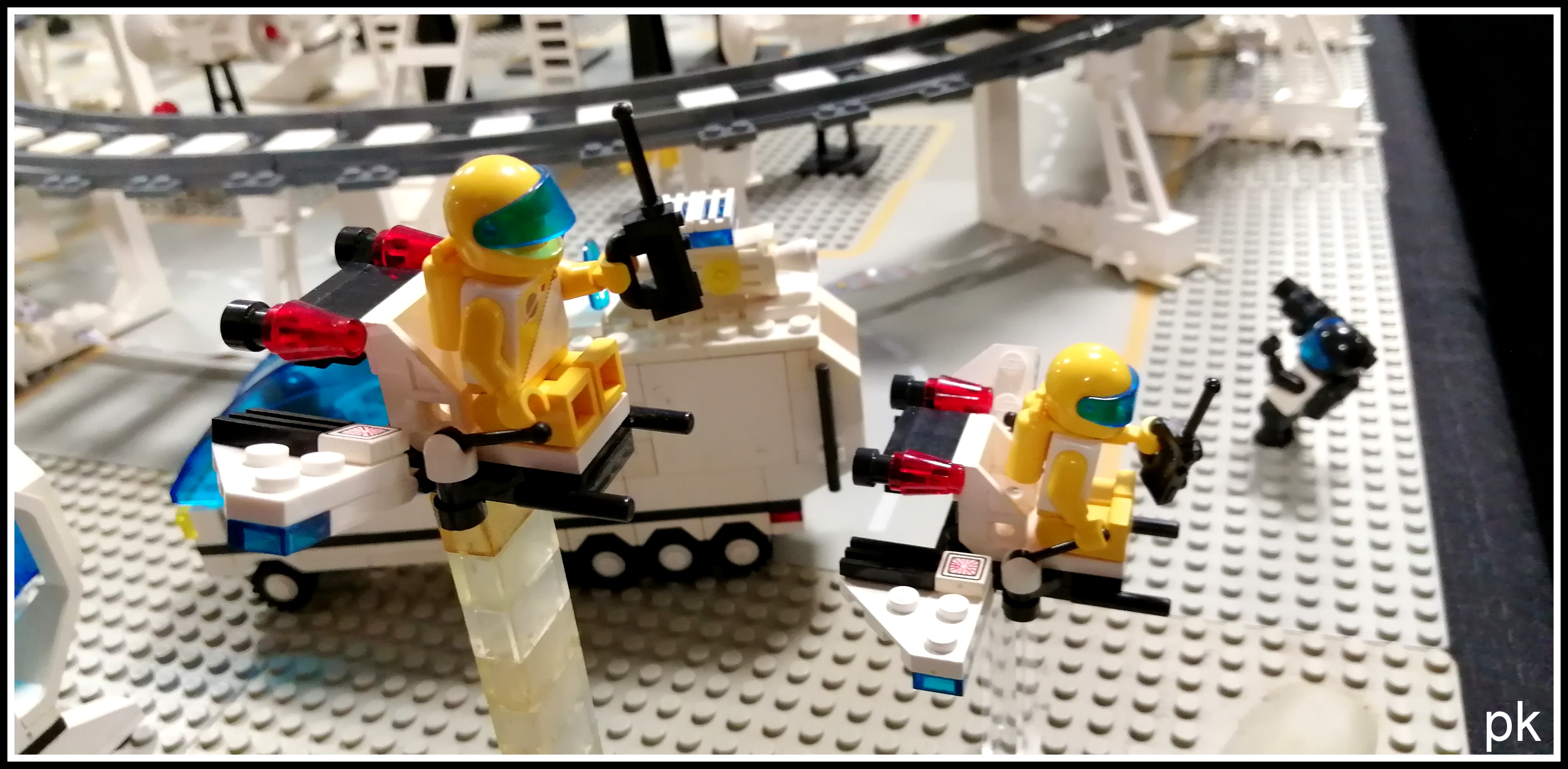This photograph captures a detailed Lego display showcasing a futuristic scene. Central to the display are two minifigures dressed in yellow astronaut-like uniforms. One astronaut is seated in a large, predominantly white truck that boasts intricate detailing, epitomizing advanced technology. The other astronaut is seemingly propelled into the air, creating a dynamic sense of movement and adventure. In the background, a railroad subtly adds depth and context to the scene, hinting at an expansive environment beyond the foreground action. Additionally, a third figure is visible, leaning backward, which further enriches the tableau with a sense of interaction and narrative. A watermark with the initials "PK" can be seen, suggesting the possible authorship of this meticulously crafted and visually engaging display.